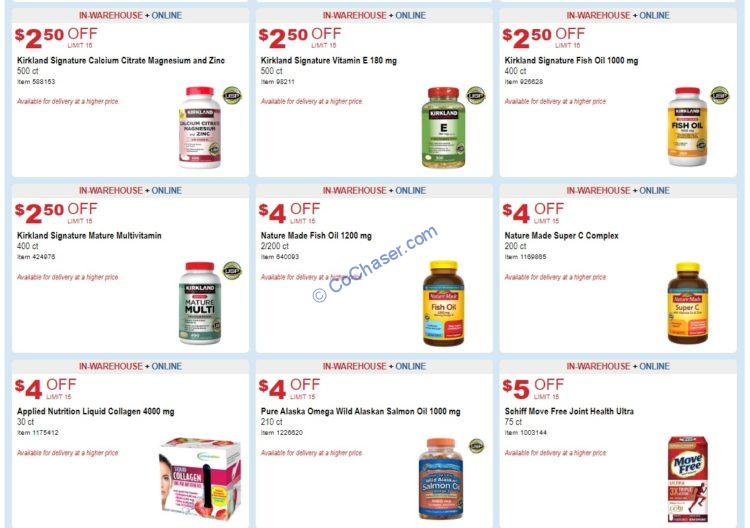Here is a polished and detailed description of the caption for the image mentioned:

---

The image showcases various discounts on a selection of dietary supplements. Featured prominently are several Kirkland Signature products:

- **Kirkland Signature Calcium Citrate Magnesium and Zinc** with a discount of $2.50.
- **Kirkland Signature Vitamin E** also discounted by $2.50.
- **Kirkland Signature Fish Oil**, available at $2.50 off its regular price.
- **Kirkland Signature Mature Multivitamin**, which has a $2.50 discount.

Additionally, there is a promotion for **Nature Made Fish Oil** offering a $4.00 discount. A significant markdown of $1200 off is highlighted for a product called **Milgram’s**, consisting of two 200-count bottles. Notably, **Nature Made Super Seed Complex (200 count)** is available for $1.50 off.

The bottom left corner of the image details a $4.00 discount on **Applied Nutrition**, which delivers 4000 milligrams. **Pure Alaska Makeup Wild Alaskan Salmon Oil (1000 milligrams)** is another featured item, depicted as a bottle of pills. 

To the right, the image presents **Phyto-Lyme 15-shift**, along with **Moo-Free Joint Health Ultra**, emphasizing its moo-free nature.

The image includes a watermark from COCHASER.COM, indicating the source of the compiled discounts and offers.

---